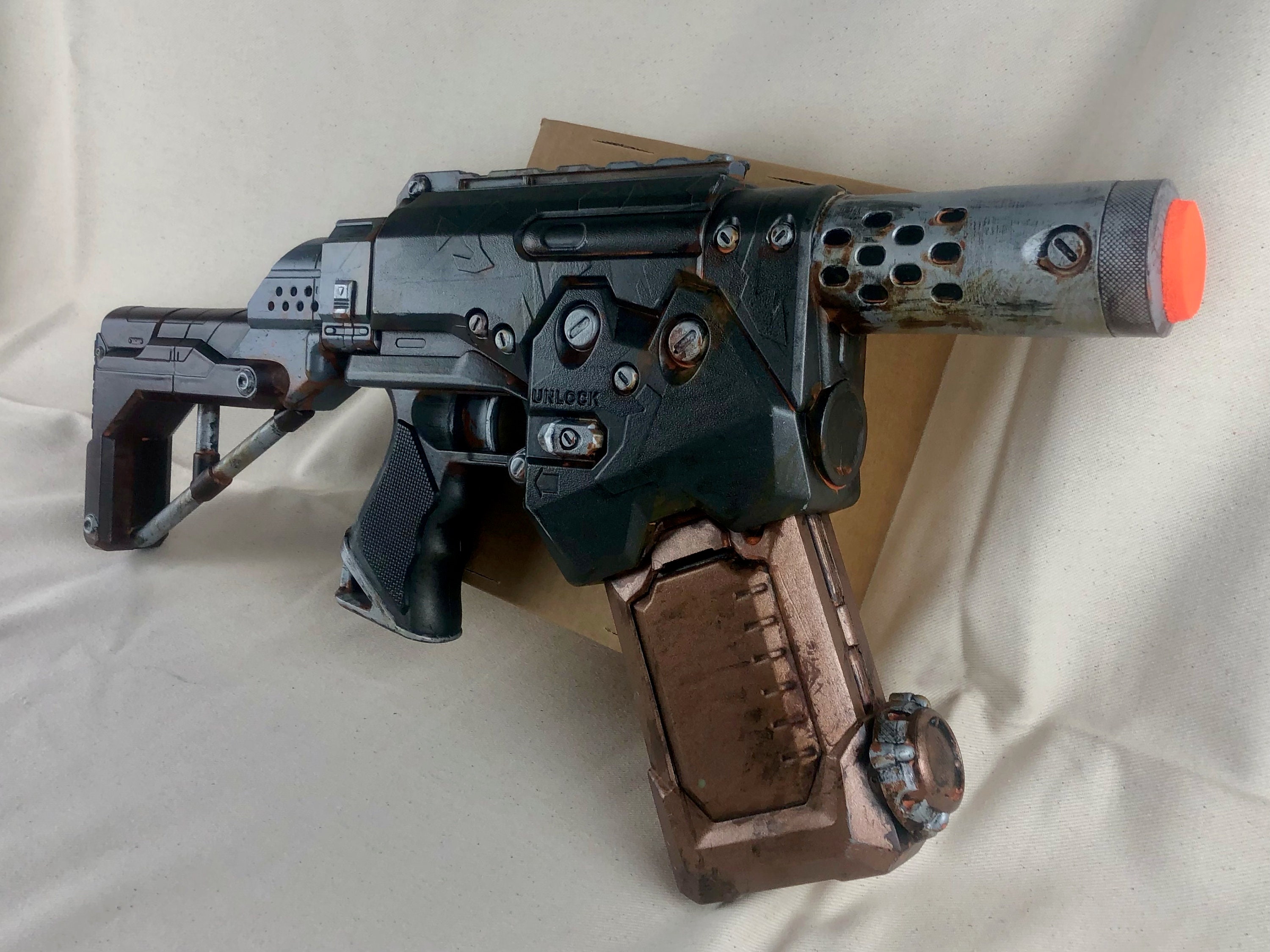This photograph captures a detailed image of a blocky toy gun, likely an airsoft or cap pistol, displayed against a white, wrinkled cloth background that resembles a bed sheet. Behind the gun, there is a brown, cardboard-like slab. The gun is quite large and predominantly black, featuring a shiny handle and a shoulder stock. Prominent features include a bronze, shiny, rectangular ammunition magazine at the front, and a short, silver barrel with an orange tip, indicative of a toy. The barrel has several rust spots and holes, with a bright yellow circular object inside. Near the back of the gun, there are dark brown rectangular components with silver tubes emerging from them. Engraved on the gun are small words, "unlock," accompanied by an arrow pointing to the left.